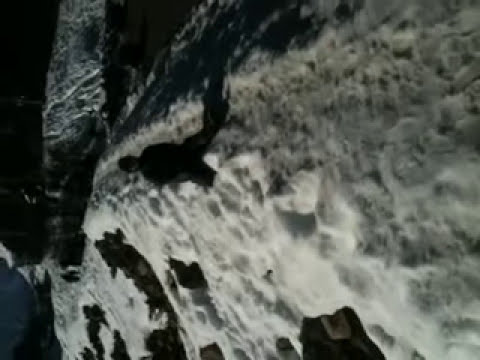This black-and-white photograph captures a scene that is open to interpretation due to its blurred and grainy quality. From behind tree branches, you can just make out a cascading waterfall in the distance. The white water sharply contrasts with surrounding dark, granite rocks that exhibit intricate gray and white patterns. In the foreground, a large pine tree looms, its needles framing the top part of the image, while a fallen tree stretches across the scene close to the waterfall itself. Adding to the depth, a tree stump sprouts from the ground on the left side of the photo. Viewed from a particular angle, the image may appear rotated, revealing a blurred silhouette of a man seemingly kneeling in either snow or water, with a snowy mountain range or more water in the hazy background. The photograph’s monochromatic palette of blacks, whites, and grays enhances its mysterious and haunting ambiance, leaving much to the imagination.